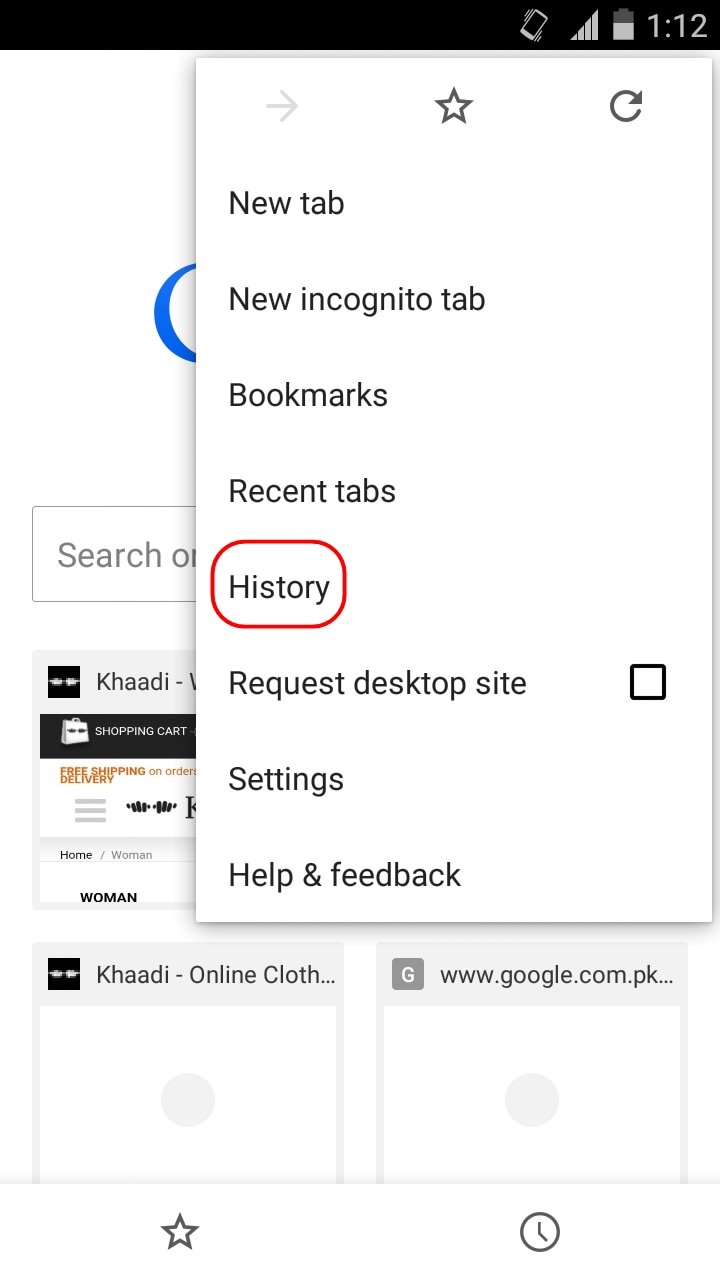A vertically-oriented rectangle image appears to be taken from a mobile device, likely a cell phone or tablet. At the very top of the image, a black bar stretches horizontally from left to right, displaying various status icons on the upper right-hand side. These icons include a vibrating phone icon, a signal strength indicator showing four bars, a battery icon displaying just over half charge, and a clock displaying the time as 1:12. Below this black bar, a white pop-up menu from the Chrome browser overlays the screen. This menu contains icons for navigation, including an arrow pointing to the right, a star, and a refresh symbol, followed by text options: "New tab," "New incognito tab," "Bookmarks," "Recent tabs," "History" (which is circled in red), "Request desktop site," "Settings," "Help," and "Feedback." The background behind this menu appears to be a white page, likely a Google search page, with a partially visible search box that is somewhat obscured by the Chrome menu.